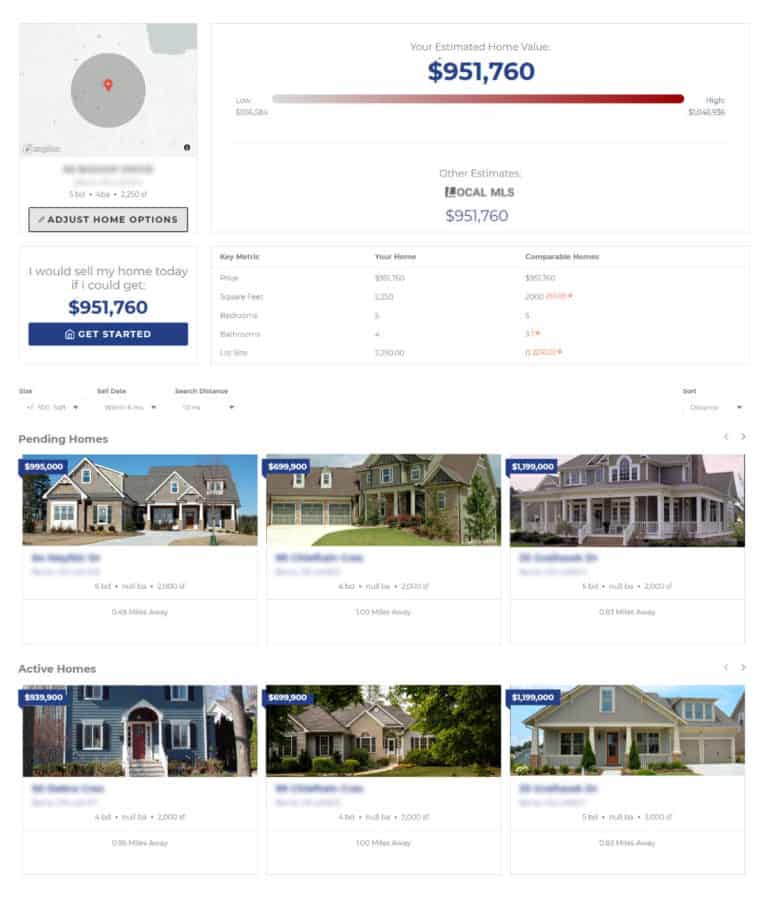A clean and detailed caption for this image could be:

"This webpage features a minimalist design with a completely white background. At the top, prominently displayed, is the target selling price of $951,760, accompanied by a sliding scale that transitions from gray to red, possibly indicating price intensity or market competitiveness. The main focus of the page is on real estate, specifically highlighting the sale of a home. Below the price, a series of small thumbnail images showcase various houses and their respective prices, likely for comparative analysis. Additionally, there is a map indicating the location of the property for sale. Some sections of the page, such as other statistical details, appear blurred out. The assortment of listed houses at the bottom serves as benchmarks to help determine a suitable asking price for the home being sold."